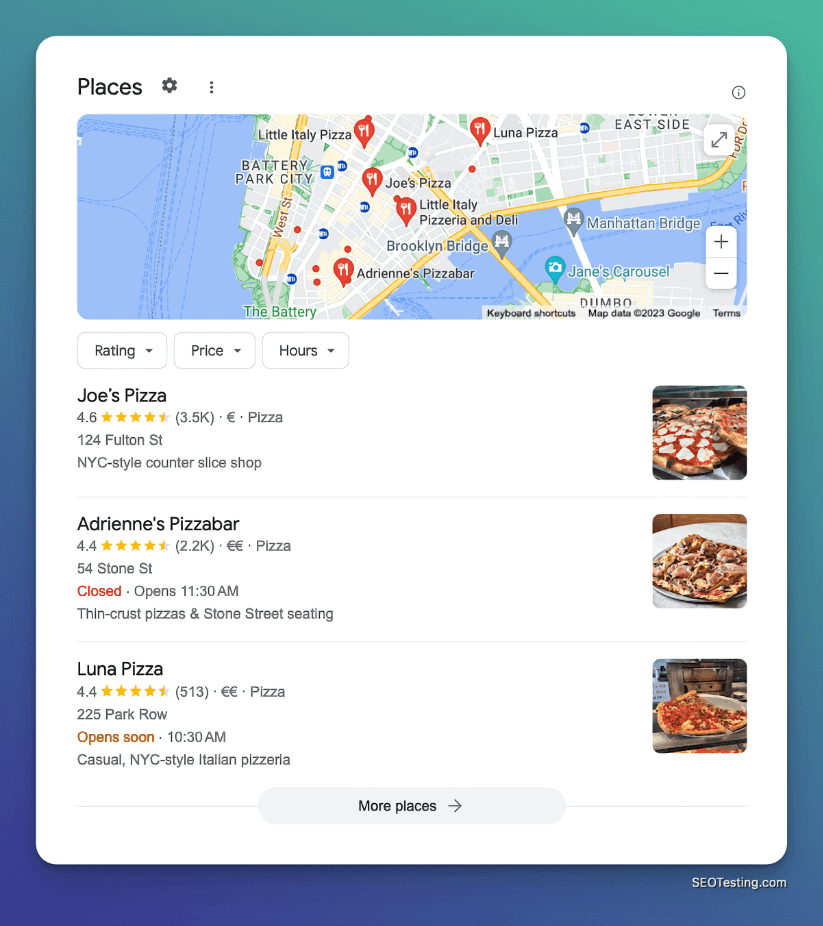The image depicts a vertically elongated rectangle with a gradient background transitioning from teal at the top to dark blue at the bottom. In the bottom right corner of this rectangle, the text "seotesting.com" is inscribed. Superimposed on this background is a smaller white rectangle, allowing a thin border of the gradient rectangle to be visible around its edges.

The white rectangle houses a header labeled "Places," accompanied by a settings icon and a vertical ellipsis (three dots). Below this header, there is another horizontally elongated rectangle containing a map with five pinned locations marked as restaurants. Underneath the map, there are dropdown menus labeled "Ratings," "Price," and "Hours."

The listings include:
1. **Joe's Pizza**: Rated 4.5 stars with 3,500 reviews, denoted by a single Euro sign indicating its price range. Located at 124 Fulton Street, it is described as a New York-style counter slice shop.
2. **Adrian's Pizza Bar**: Rated 4.4 stars with 2,200 reviews, marked by two Euro signs to indicate a higher price range. It is situated at 54 Stone Street and is currently closed, with plans to open at 11:30 AM. The description highlights thin crust pizza and street seating.
3. **Luna Pizza**: Specific details about Luna Pizza are not fully provided in the description.

Each entry includes the restaurant name, rating, number of reviews, price range, address, and a brief description of the establishment.